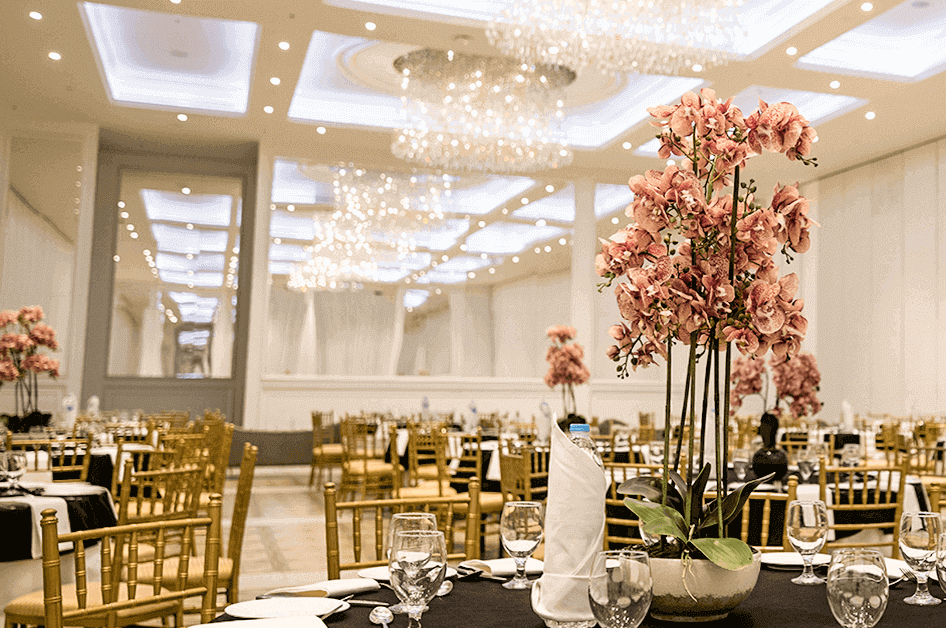The image showcases a lavishly decorated event hall, likely prepared for a wedding. The room is illuminated with radiant white lights from glass chandeliers and recessed ceiling fixtures, giving it a bright and elegant ambiance. The space features gold chairs surrounding tables draped in black and white linens. Each table is meticulously set with unused white plates, cutlery, and both wine and water glasses. Prominently, each table displays a light pink floral centerpiece in a white and black bowl, accented with green leaves. Decorating these tables are also napkins, some elegantly placed in coffee cups. The room's walls have hints of grey, adorned with large mirrors, and a divider creating an impression of multiple rooms. In addition to this, white drapes cascade down in the adjacent area, enhancing the hall's sophisticated decor.